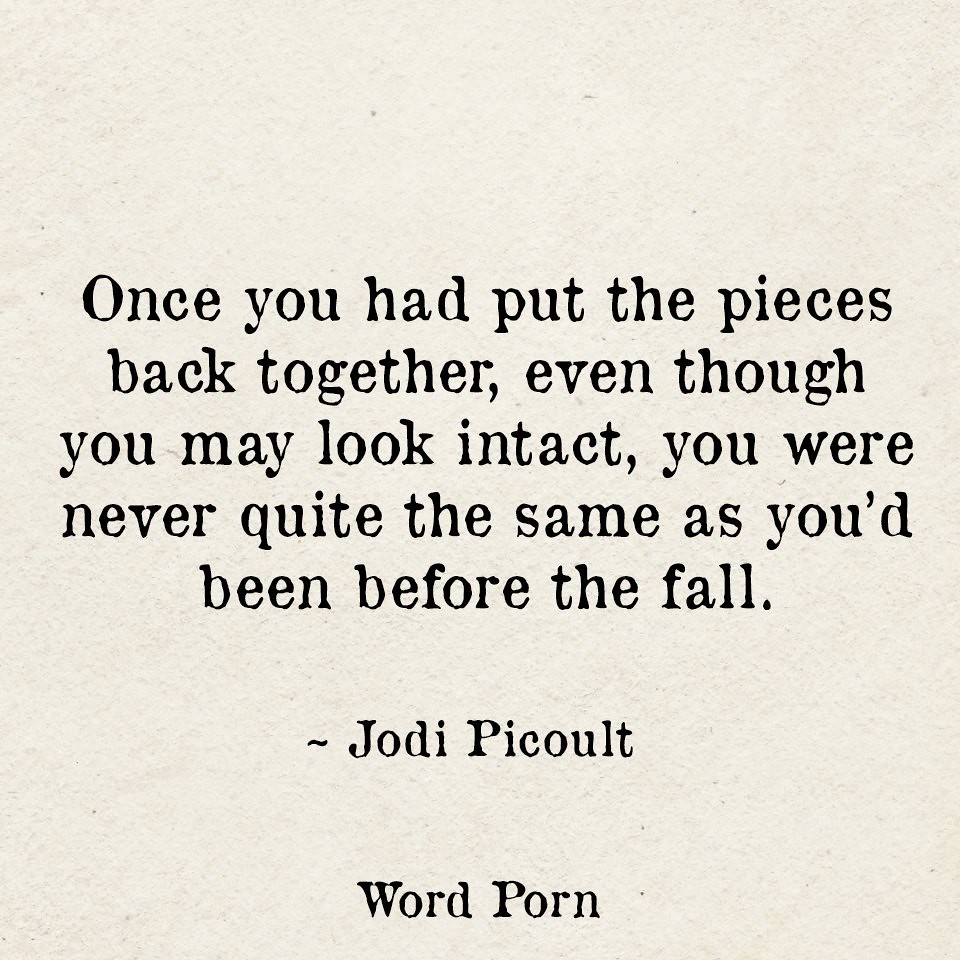An inspirational quote, presented on an off-white, slightly pinkish textured paper, is centered in the middle of the image in a classic black font reminiscent of an old typewriter. The quote reads, "Once you had put the pieces back together, even though you may look intact, you were never quite the same as you'd been before the fall." Below the quote, there's a small dash mark followed by the author's name, "Jodi Picoult." At the very bottom of the image, the phrase "Word Porn" is subtly printed, adding a final touch to the overall minimalist design.